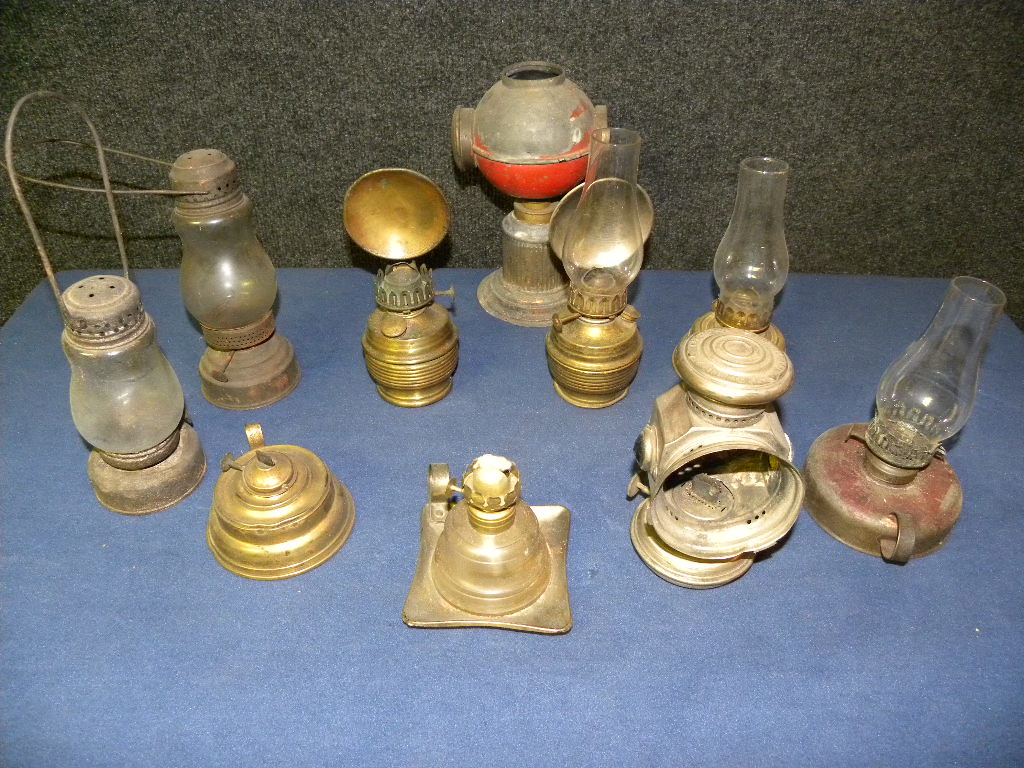This image depicts a collection of antique oil lamps and lanterns, displayed on a weathered, blue-gray table against a grainy charcoal gray wall. The assortment includes ten varied lamps, some resembling traditional ship lanterns. Many of these lamps are incomplete, missing parts such as glass components and hurricane lamps. They exhibit significant signs of wear and tear, with weathered and rusted surfaces, tarnished brass, and faded paint. Notably, a large, chipped red lantern stands out in the back, missing its hurricane lamp. The glass elements, where present, appear foggy and dirty, contributing to the overall rustic and historical aesthetic of the scene.